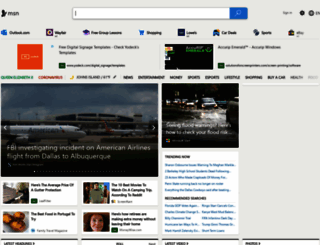The image is a detailed screenshot of a webpage, presumably from MSN. At the top, there is a search bar with a blue square containing a white magnifying glass icon, indicating the search functionality. Below the search bar, there is an orange square and a black rectangle, both containing some form of additional information.

Prominently displayed in the center of the page is an image of an airplane at an airport, with a headline that reads: "FBI Investigating Incident on American Airlines Flight from Dallas to Albuquerque." Just below this main headline, there's another image depicting cars on a street, partially overlaid with white text that is difficult to discern from the screenshot due to its small size. The section is labeled "Trending Now" with additional text in blue, presumably hyperlinks to other trending articles.

Further down the page, there are four smaller articles. The first of these articles features an image of a woman, suggesting that the story may revolve around her. The exact details of the articles and images are not completely clear from the description but the layout and elements suggest a typical news webpage with headline stories and trending topics.